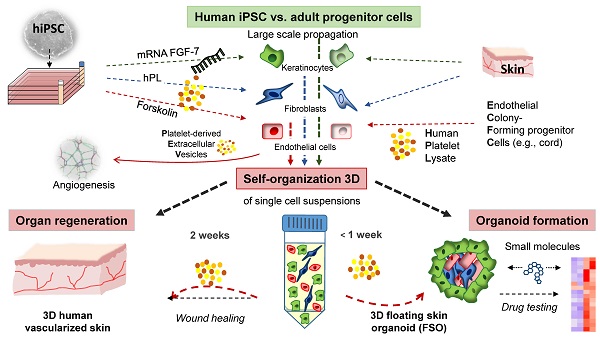The diagram depicts various processes and components involved in the cultivation and application of human iPSC (induced pluripotent stem cells) versus adult progenitor cells. The background is solid white, and it features several detailed sections:

At the top, a green rectangle with black text reads "human iPSC versus adult progenitor cells." Directly below this, the term "large scale propagation" is highlighted, with icons beneath it including green dotted arrows pointing to different segments. One arrow directs towards a pink icon labeled "skin," while another points to an illustration resembling a boxing ring with a gray circle labeled "HIPSC," accompanied by a downward arrow.

In the middle section of the diagram, a red-background rectangle is labeled "self-organization 3D." Underneath this, the text specifies "single cell suspensions." Below this label, there's an illustration of a bottle with a blue cap and pointed bottom containing molecules depicted in green, red, and blue.

Additional details include icons and arrows representing various cell types, such as keratinocytes, fibroblasts, and endothelial cells, indicating their roles in processes like organ regeneration and wound healing. The diagram also features concepts like "3D human vascularized skin," "3D floating skin organoid," and "small molecules and drug testing," illustrating the potential applications of these cells in medical treatments.